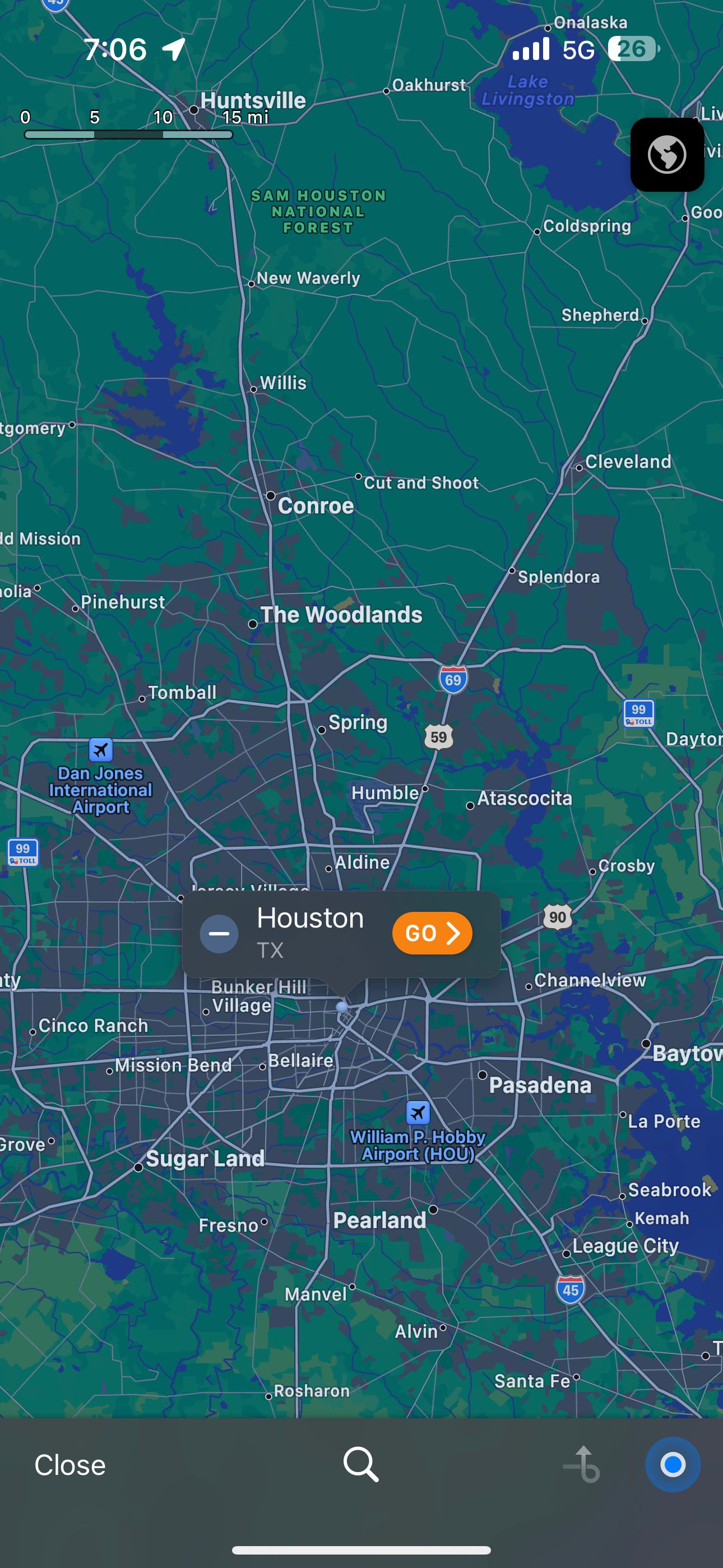This image displays a screenshot from a non-Google maps application on a mobile phone, showcasing a detailed satellite view of Houston, Texas, along with its neighboring cities and suburban areas within the county. Centrally positioned on the map is a gray speech bubble, prominently displaying "Houston, Texas" in white text. To the left of this label is a gray circle containing a minus sign, while to the right is an orange bubble with the text "Go."

The map highlights significant areas around Houston, including the downtown region, the Woodlands, and major highways such as Interstate 69. Additionally, it features the Sam Houston National Forest situated to the north of Houston and Lake Livingston located to the northeast.

At the top of the screenshot, several pieces of information are displayed: the phone is connected to a 5G network and has 26% battery remaining. The current time, 7:02 PM, is shown in the top left corner.